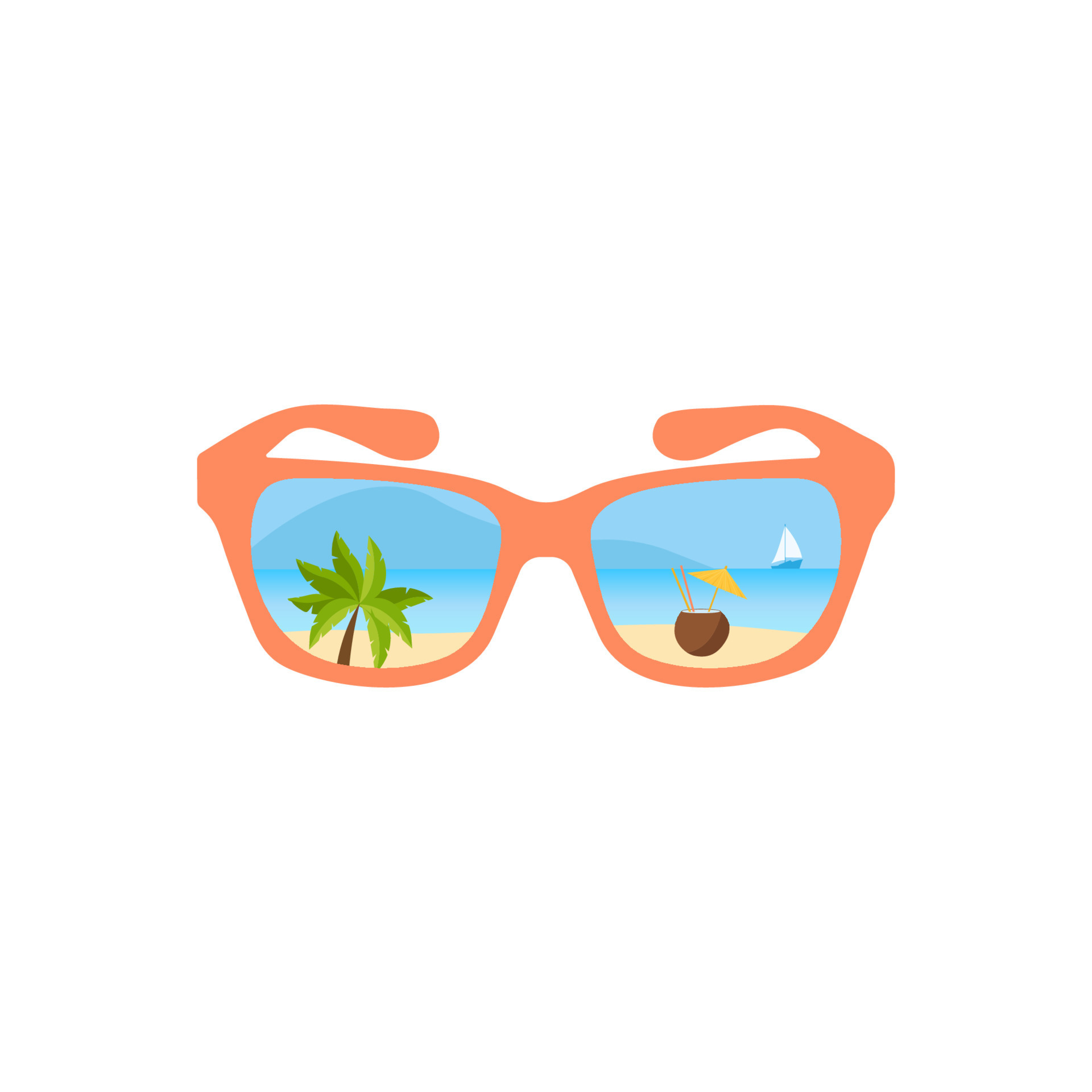The image is a simplistic piece of vector art showcasing a pair of clip art sunglasses against a completely white background, which occupies the majority of the space. The sunglasses are peach-pink or orange in color and are positioned so that you are looking straight at the lenses, with the ear pieces extending backward. The lenses artistically depict a vibrant beach scene. In the left lens, there's a palm tree with alternating light and dark green leaves, sandy beach, blue ocean waters, a distant mountain silhouette, and a boat sailing in the water. The right lens features light sandy beach with a cut-open coconut, adorned with a yellow umbrella and wooden straw, set against the expanse of the ocean and a blue sky. The beach scene's intricate details include the inviting blue hues of the ocean and the sky, enhancing the overall summery and tropical theme.